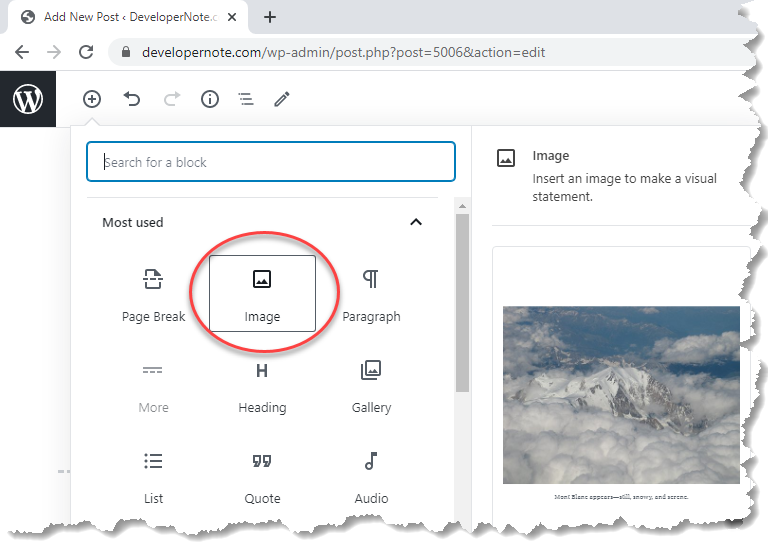This screenshot captures a detailed view of a computer desktop, specifically on a laptop or desktop computer, showcasing a web page open to a post editor. The browser tab, located at the top, displays a globe icon and the partial title "Add New Post - Developer Note.com," accompanied by the standard tab controls such as an "X" to close the tab and a "+" to open new tabs. A light gray navigation bar runs across the top of the screen. 

The overall image is rectangular, with the bottom and right edges made to appear as if they are torn paper, complete with a gray shadow underneath these jagged edges, enhancing the effect. Below the navigation bar, we see typical browser buttons: a left-facing arrow for back navigation, a refresh arrow, and a search bar showing a secure web address: "developernote.com/wp-admin/post.php?post=5006&action=edit". Next to this URL is a lock icon, indicating a secure connection.

On the left side of the view, there's a black square with a white "W" inside a circle, likely representing the WordPress logo. Moving right from this icon, there are several tools: a "+" icon for adding elements, a back arrow for undoing actions, followed by a grayed-out redo arrow, indicating no actions have been performed yet. There's also an information button, a three-line menu icon, and a pencil icon for editing.

Below this toolset, a search bar invites users to "Search for a block." Directly underneath it, there's a list titled "Most Used," featuring options like "Page Break," "Image," "Paragraph," "More," "Heading," "Gallery," "List," "Quote," and "Audio." Notably, someone has highlighted the Image option using a red oval shape. 

On the right side, there's a detailed section concerning images. It displays the word "Image" with an icon that allows users to add additional photos. Text underneath reads, "Insert an image to make a visual statement." In the bottom right corner of the screen, there's a photograph of snowy mountain peaks emerging above a blanket of clouds, suggesting the photo was taken from an elevated vantage point, likely from an airplane or helicopter. Below the photograph, there appears to be some unreadable text.